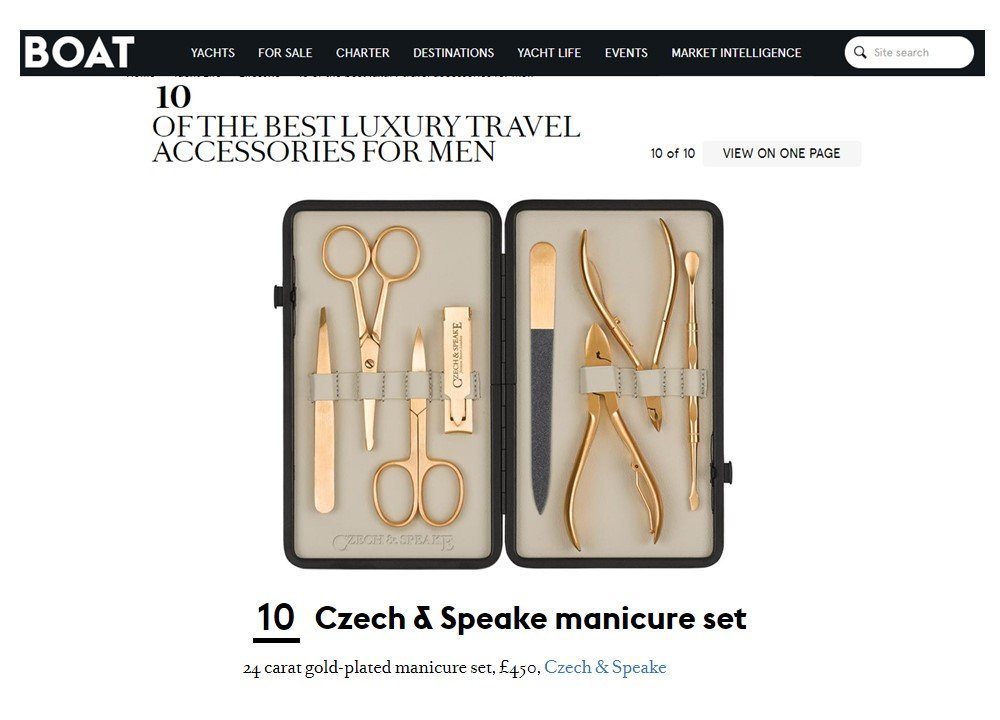The image features a webpage showcasing a luxury product advertisement for the "Check and Speak" 24-karat gold-plated manicure set. At the top left corner of the webpage is the "boat" logo in white text, next to a horizontal navigation bar with options including "Yachts for Sale," "Charter," "Destinations," "Yacht Life," "Events," and "Market Intelligence." On the far right is a search field labeled "Search Site." The body of the page prominently displays the headline, "10 of the Best Luxury Travel Accessories for Men," indicating this is item 10 out of 10 in the list.

The featured manicure set is housed in a sleek black case with a tan interior. The set includes various grooming tools, all with a luxurious rosy gold finish. These tools comprise tweezers, two pairs of scissors, nail clippers, a nail file with a black filing surface and gold handle, two nippers, and a cuticle tool. The bottom of the webpage further details the product as the "Check and Speak Manicure Set," priced at £450, emphasizing its 24-karat gold plating.